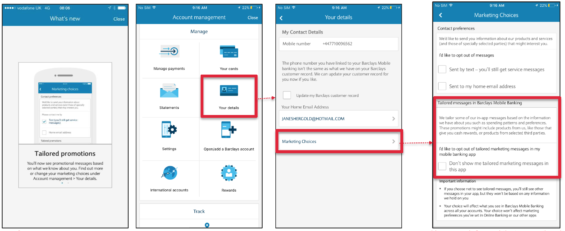This image features a composite of four mobile webpage screenshots, each bordered by a blue header. The first screenshot displays a webpage with a centered pop-up box. The header reads "What's New" in the center, with a "Close" button to the right. Inside the pop-up box at the bottom, it states "Tailored Presentations," followed by a brief description. A partial view of a white iPhone is visible on this page, although the image is significantly blurred, indicating that it has been enlarged and lost its clarity.

The second screenshot, titled "Account Management," features one option highlighted in a red box. A connecting arrow leads from this red box to a similar red-boxed option on the third screenshot. The third screenshot continues the sequence with another red-boxed option, from which an arrow leads to the fourth screenshot. The fourth screenshot's header reads "Marketing Choices," and a large red box encircles text in the middle. However, due to the extreme blurriness of all the screenshots, the text within the red boxes, especially in the fourth image, is illegible.